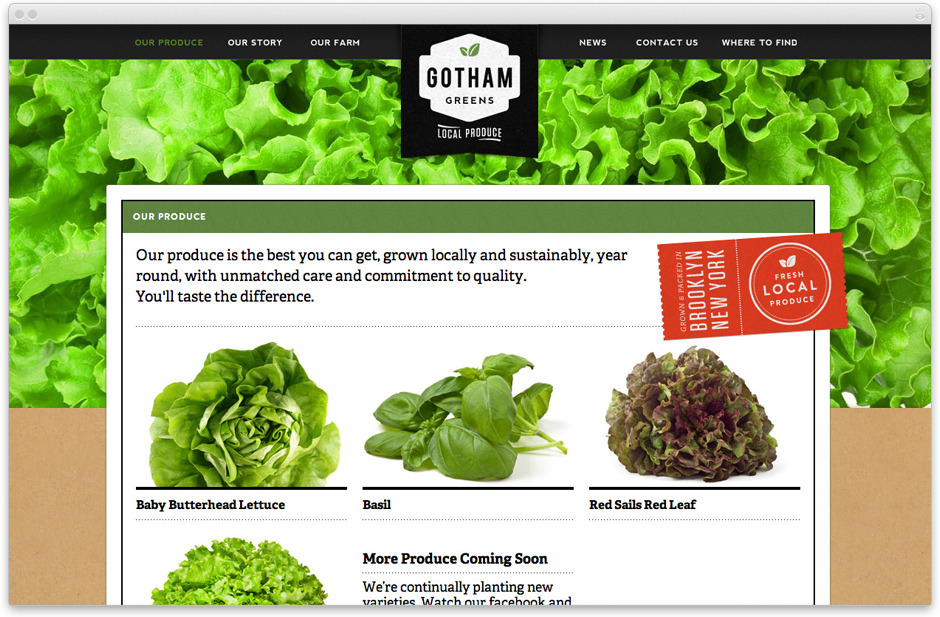This image appears to be a detailed screenshot of a homepage for Gotham Greens, a prominent produce producer. The web page is presented on a clean, white background that frames the content. The header section of the webpage features a vibrant green leafy lettuce, creating an eye-catching and fresh look. Just below this verdant imagery, a brown section evokes the texture and color of a shopping bag, symbolizing the natural and fresh nature of the produce being offered.

At the very top of the page, a black-colored menu bar lists navigation options in green text, including: "Our Produce," "Our Story," "Our Farm," "News," "Contact Us," and "Where to Find." Central to the page’s design is the Gotham Greens logo, which is stylized within a hexagonal shape. The logo prominently features the brand's name in black text, two green leaves above it, and the phrase “Local Produce” in white just beneath it.

Directly below the header, there is a green bar on the left side with white text that reads "Our Produce." Adjacent to this bar, a describable text in black asserts: "Our produce is the best you can get, grown locally and sustainably year-round with unmatched care and commitment to quality. You'll taste the difference." To the right of this, a red ticket icon marked with "Brooklyn, New York" in white emphasizes the local nature of the produce offered.

Further down the page, images of different types of produce are displayed. There is an image of Baby Butterhead Lettuce labeled accordingly, an image of Basil labeled "Basil," and an image labeled "Red Sales Red Leaf" for this specific type of lettuce. Lastly, a message indicates that more produce varieties are continually being planted, encouraging visitors to watch their Facebook page for updates.